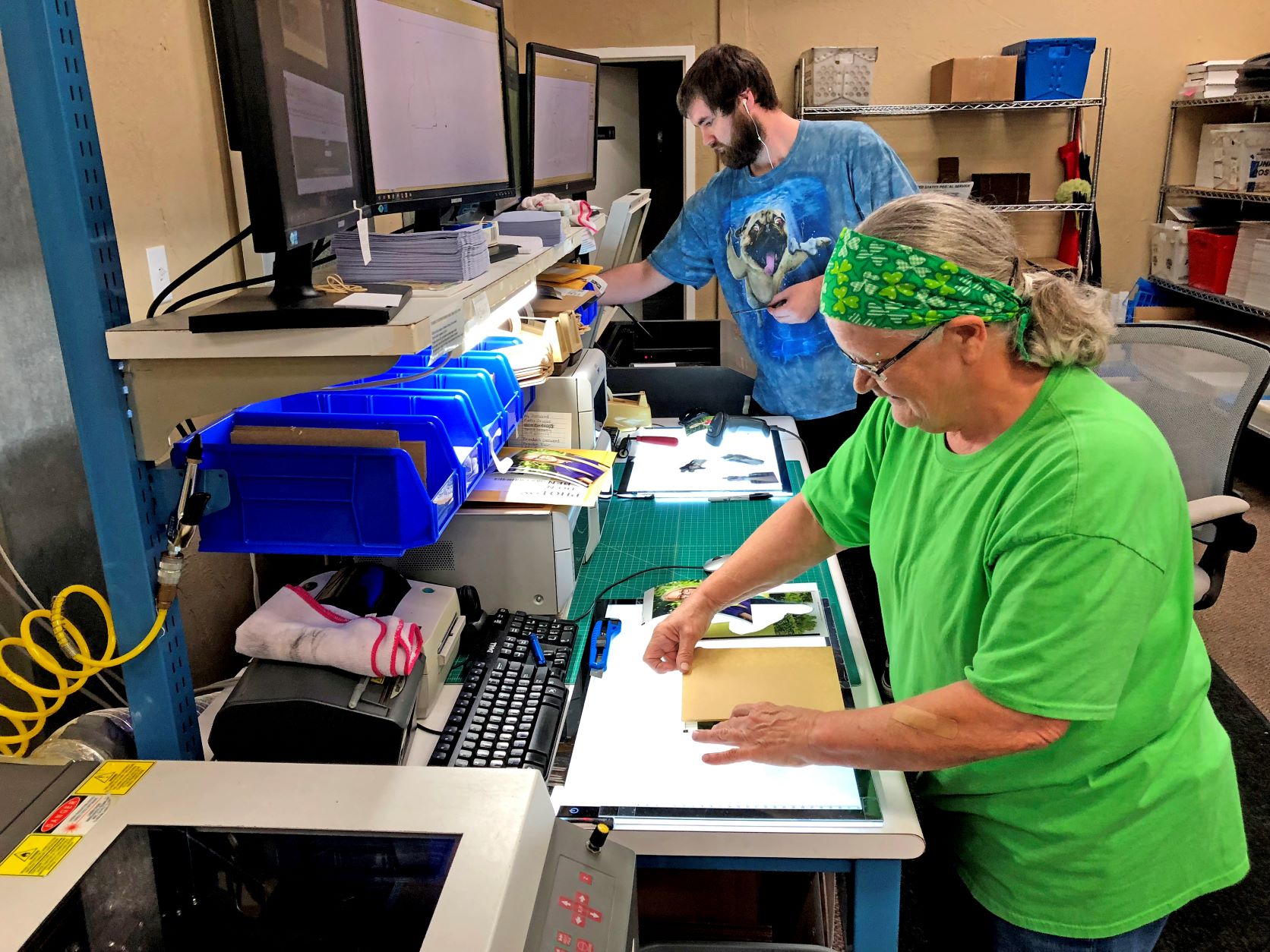In this detailed and dynamic image, two individuals are collaboratively working on a project involving physical prints in a well-organized workspace. On the left, a complex setup of a copier with wires feeds into a set of tubes connecting to blue tubs brimming with artistic materials. Underneath these tubs, a keyboard and a couple of printers can be seen, while another level of shelving above holds three monitors displaying essential information. 

On the table in the foreground, two white canvas boards are brightly lit and carefully measured. The woman, engrossed in her task, wears a vibrant green t-shirt and a shamrock-adorned bandana that holds her hair back. Her glasses reflect her concentration. To her right, a man is seen wearing a blue t-shirt featuring a pug dog swimming towards the viewers. He has dark brown hair, a substantial beard, and an earbud in his left ear, likely listening to something privately as he works. Their seamless coordination amidst the array of screens, supplies, and artistic materials speaks to a shared dedication to their meticulous and creative endeavor.